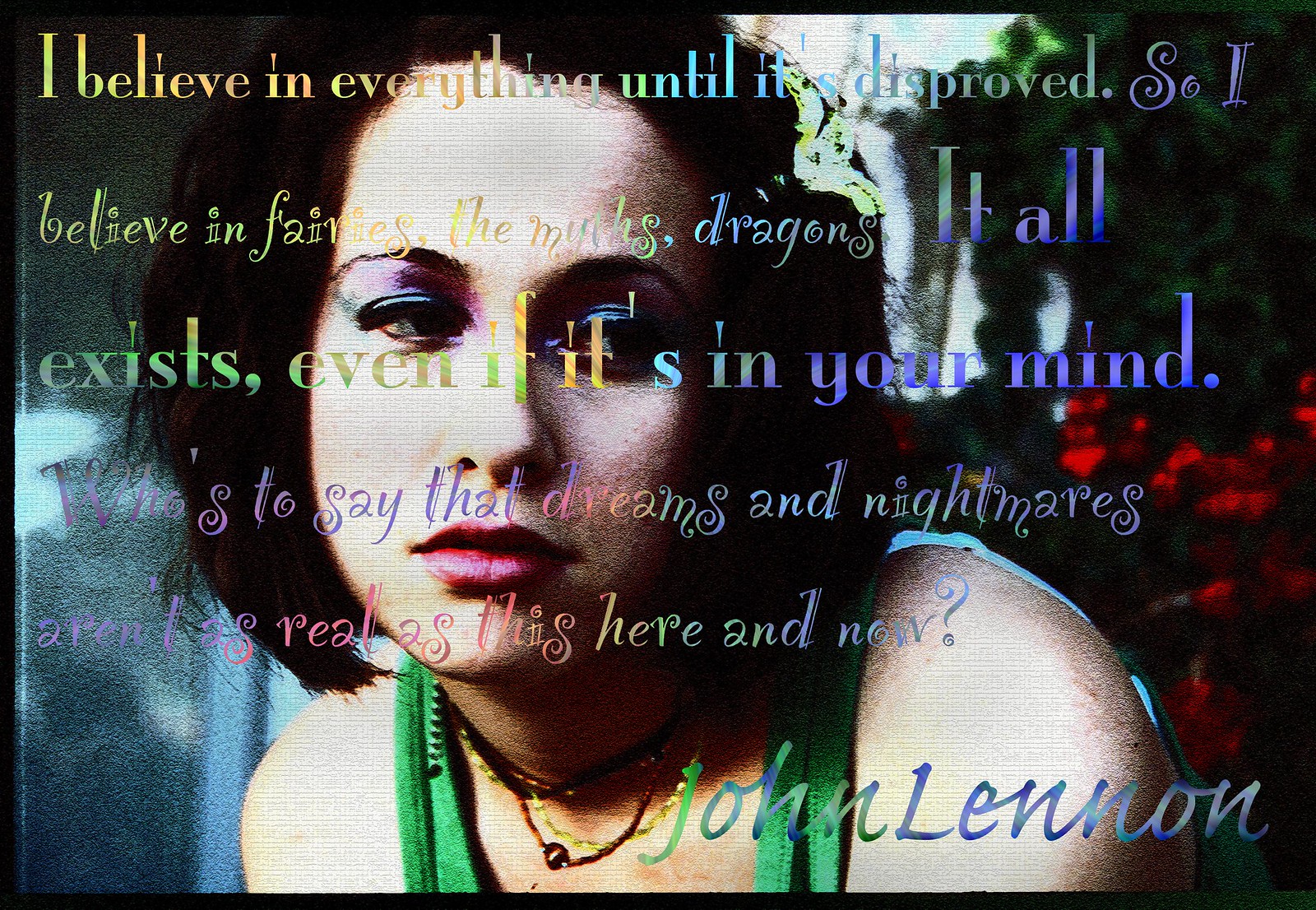The image resembles an album cover, featuring the name John Lennon at the bottom right corner. Dominating the composition is an expressive artistic filtered photo of a woman with short black, shoulder-length hair. She is wearing striking blue eye shadow or eyeliner and light red lipstick. Her gaze is directed slightly to the right, giving her a contemplative, somewhat sad look. She is adorned with necklaces, including a noticeable choker, and is dressed in a green top with straps visible over her shoulders.

Filling much of the space behind and around her are multicolored texts in various fonts, displaying a quote attributed to John Lennon. The text reads: "I believe in everything until it's disproved. So I believe in fairies, myths, dragons. It all exists even if it's in your mind. Who's to say that dreams and nightmares aren't as real as this here and now?" This text is rendered in a vibrant array of colors including purples, yellows, greens, and blues, creating a striking visual contrast against the more subdued colors of the background, which features blurred elements of green and red, possibly flowers. The entire image is framed with a black border, giving it a cohesive finish.